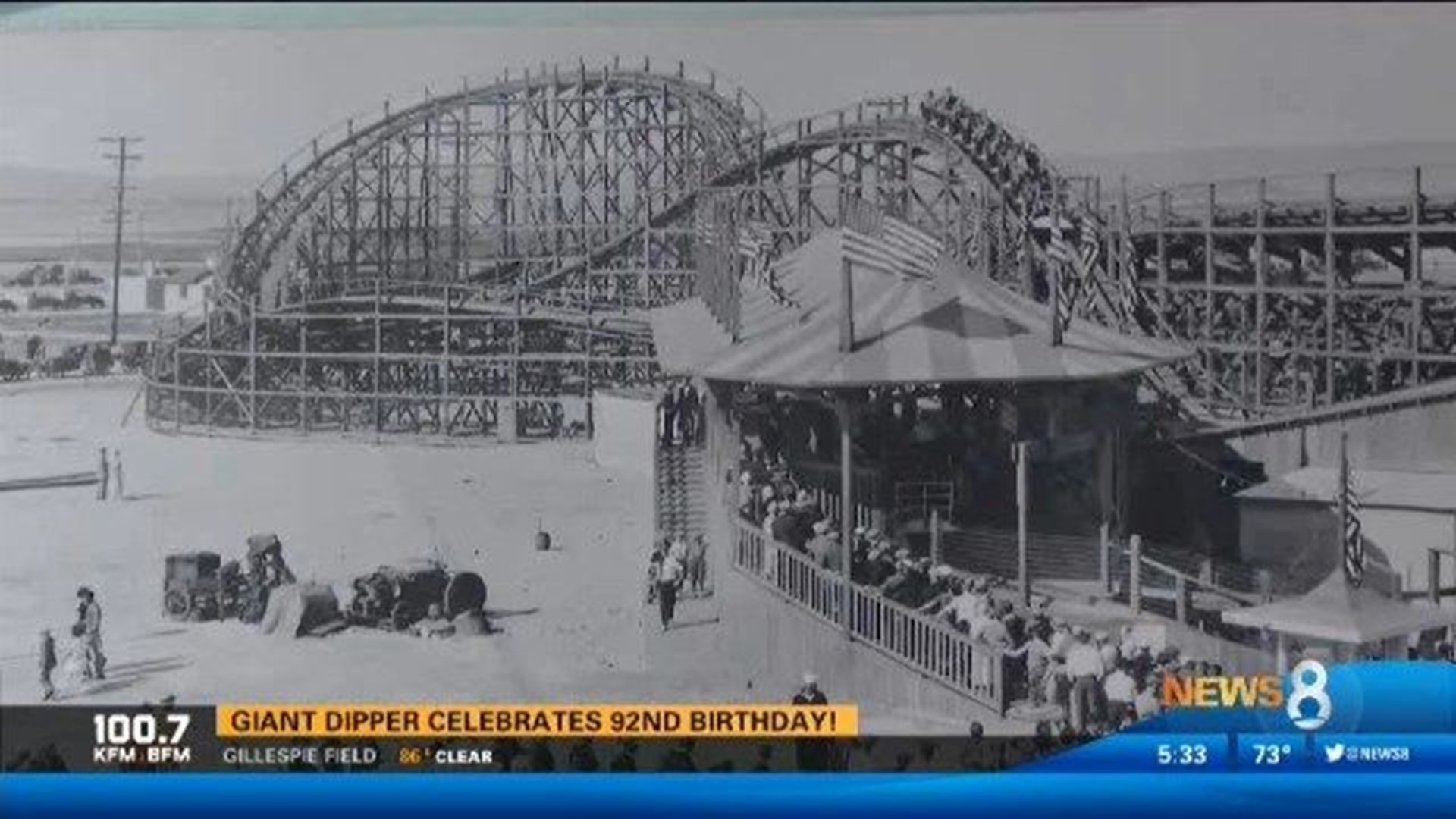This image, taken from a TV news report, features an old black and white photograph of the Giant Dipper, a wooden roller coaster celebrating its 92nd birthday. The broadcast information at the bottom of the screen includes a light blue banner displaying "100.7 KFM BFM," "Gillespie Field 86 clear," and "News 8" with the time "5:33" and "73 degrees." Above this, a yellow box with black writing announces the Giant Dipper's milestone. In the black and white photo, reminiscent of an early 20th-century amusement park scene, people dressed in period attire are seen waiting in a long line under a circus tent canopy adorned with American flags, eager to ride the historic roller coaster. The image captures not only the spirit of the era but also the significance of the Giant Dipper in amusement history.